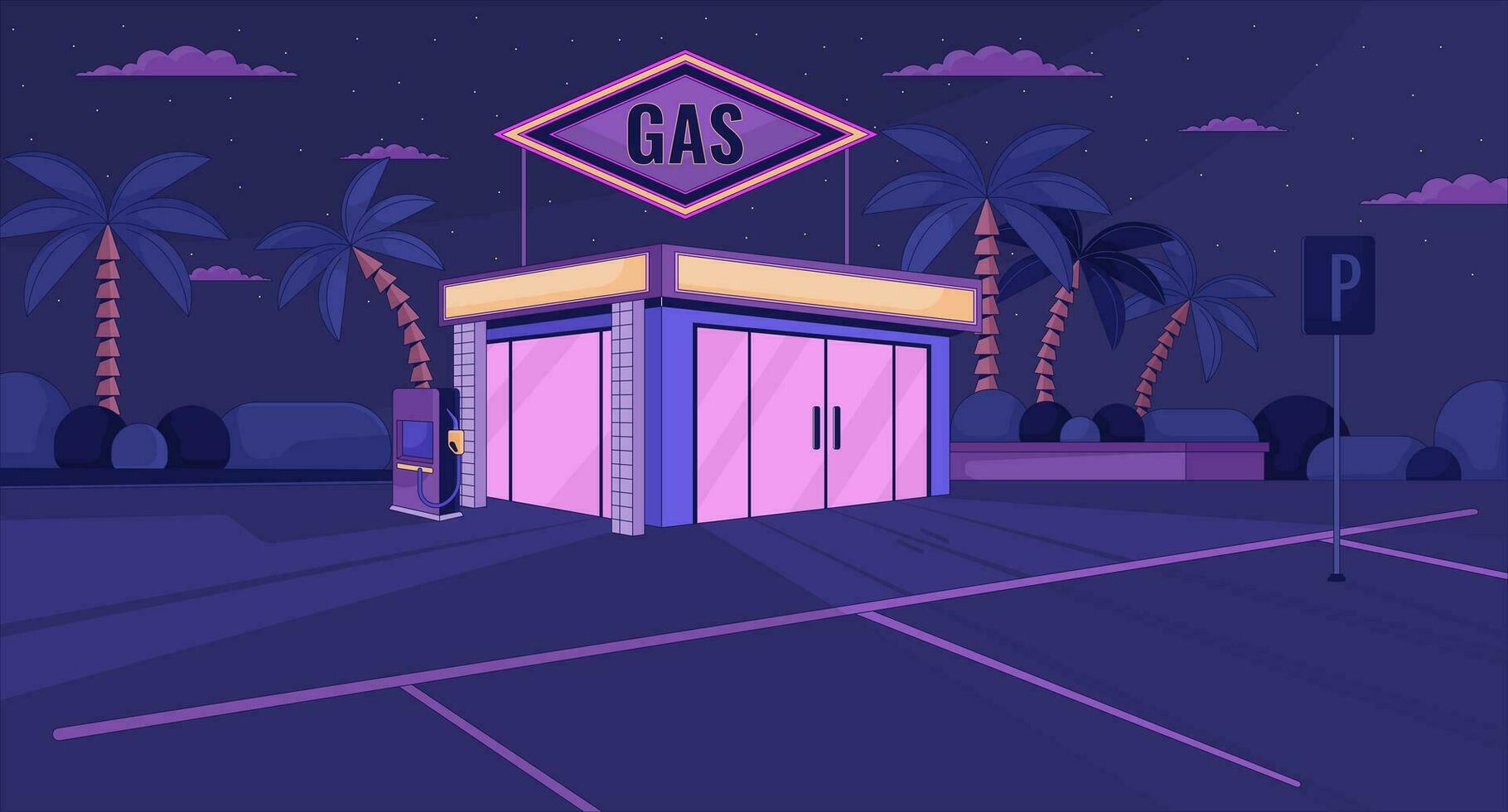This image is a detailed and colorful cartoon drawing of a gas station, reminiscent of something you might see in *The Simpsons*. The scene is dominantly hued in shades of purplish blue, with the sky, parking lot pavement, and various elements of the gas station sharing this color scheme. The gas station itself features a structure with large windows and yellow trim at the top, complementing its pink and purple facade. 

A prominent diamond-shaped sign reading "GAS" in bold black letters sits atop the building, also colored purple. A purple gas pump stands beside the store, which has a mauve front and side doors trimmed in medium blue. The parking lot is marked with purple and pink stripes, including a parking space sign distinguished by a large letter "P".

Adding to the scenery, green-leafed, brown-trunked palm trees stand behind the store, contributing to the tropical atmosphere. Interestingly, the palm trees and some clouds also show hints of pink and blue. The entire illustration gives off a vibrant, night-time feel with its rich and varied color palette, textural detail, and whimsical charm.